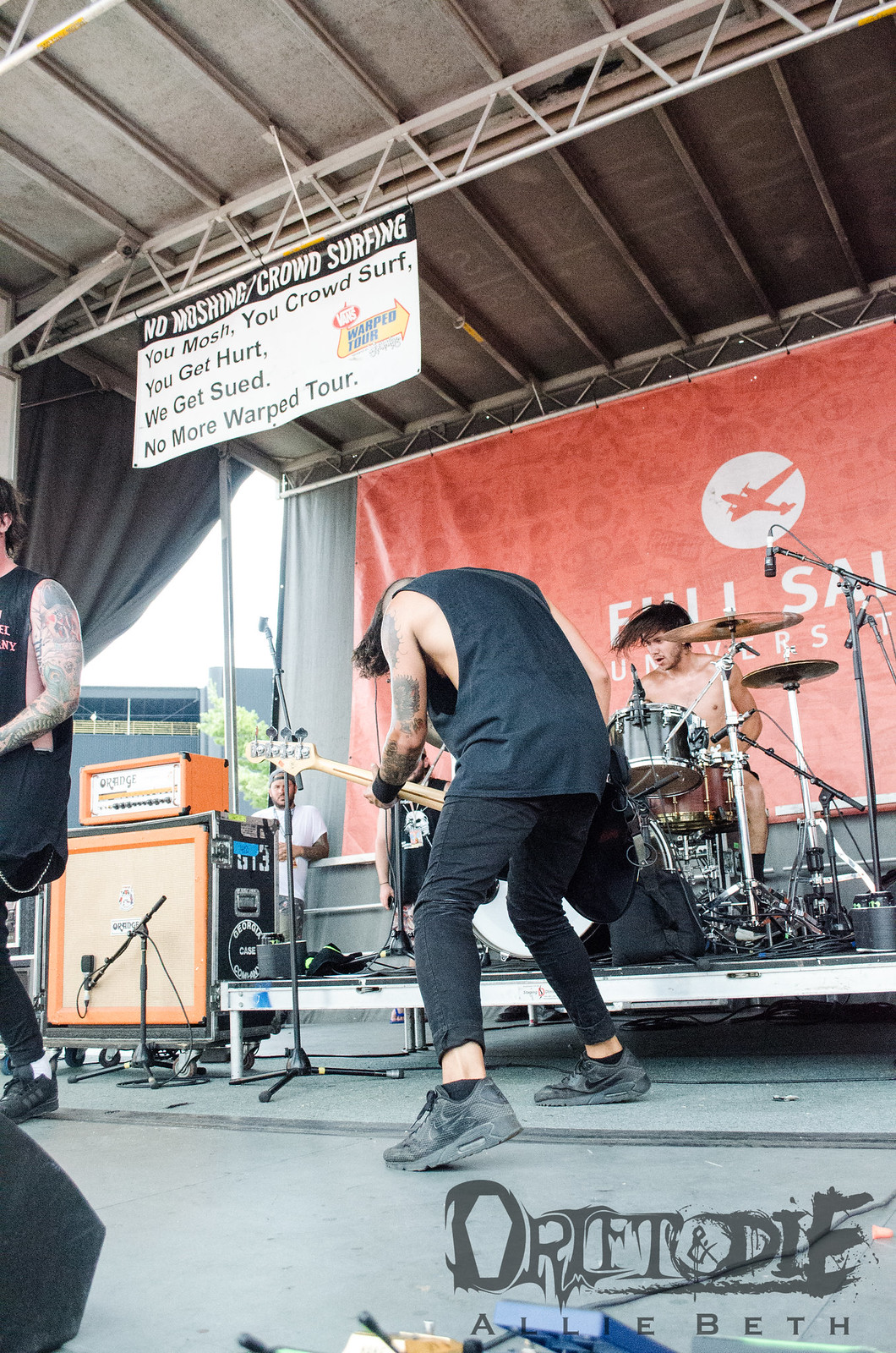The image captures a dynamic scene at an outdoor rock concert, likely during a Vans Warped Tour in the middle of the day. It is a tall, rectangular photograph featuring multiple musicians on stage. The bottom half of the image reveals a grayish-green, semi-carpeted, dusty stage surface. A platform crosses from right to left, supporting a black metallic drum set with several cymbals. A shirtless drummer with long, flying hair energetically plays in the top right corner, behind a large orange-colored poster.

In the center of the image stands a man deeply immersed in his guitar performance. Bent over and facing away from the camera, he sports a black tank top, dark brown pants (or black jeans according to another description), and black Nike Air Maxes. To his left, partially cut off, is another man with a tattooed arm; he is also dressed in black with a Muscle shirt and Adidas shoes. Above them, a sign prohibiting moshing and crowd surfing is visible, capturing the essence of the concert's lively yet controlled atmosphere. The backdrop may feature the logo of Full Sail University, adding to the contextual details of this high-energy musical event.